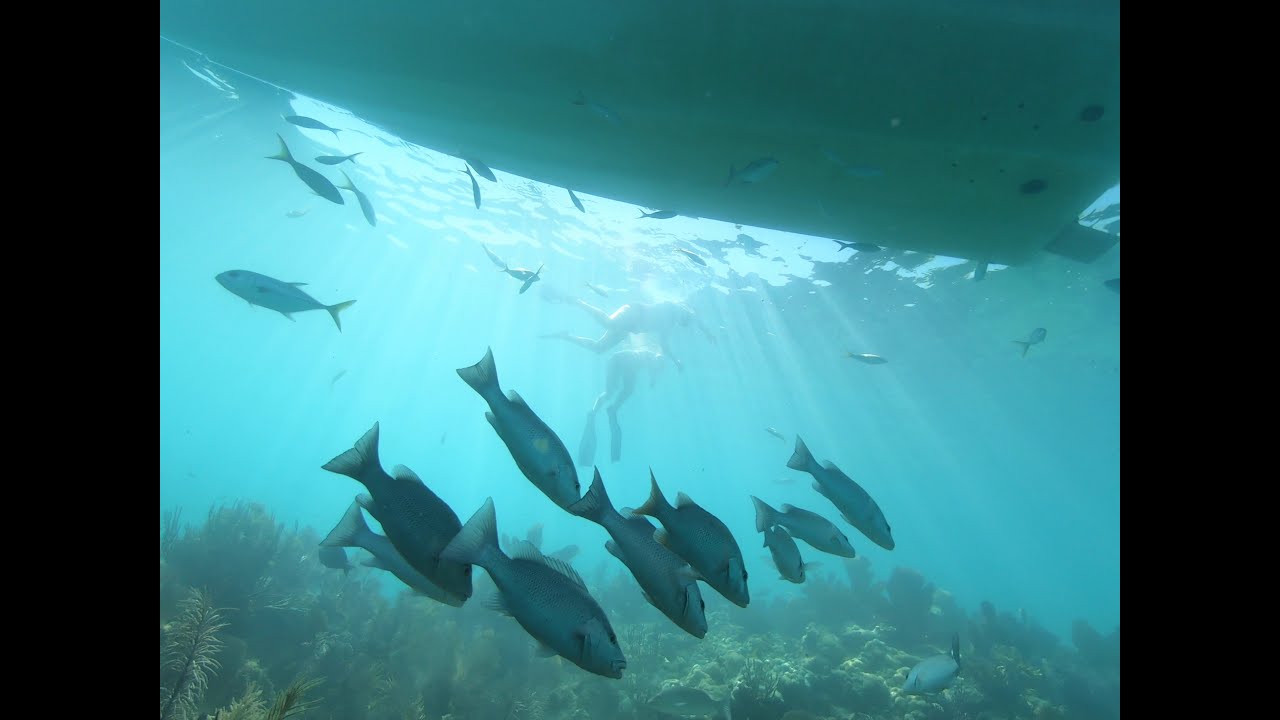This horizontally aligned rectangular underwater photograph, framed by vertical black borders on both sides, presents a surreal aquatic scene. At the top of the image, the flat, light blue bottom of a boat is visible, starting from the top left corner and curving down towards the middle of the right side, with sunlight rays penetrating the bright blue water below. Below the boat, the vibrant coral reef flourishes with green plants and algae, scattered across the ocean floor. A school of medium-sized, gray fish, characterized by lighter tails and fins, are swimming prominently towards the bottom right corner of the picture. Their metallic appearance contrasts with the traditional, dark blue hue of other species swimming in all directions throughout the scene.

In the background, the image also captures the subtle presence of two scuba divers. One diver, barely discernible, is swimming through the water, while the other hangs suspended with outstretched legs. Nearby fish, some appearing to be feeding among the coral, interact harmoniously with the divers. The entire underwater tableau is bathed in the ethereal play of light and shadow, encapsulating a moment of tranquility beneath the waves.